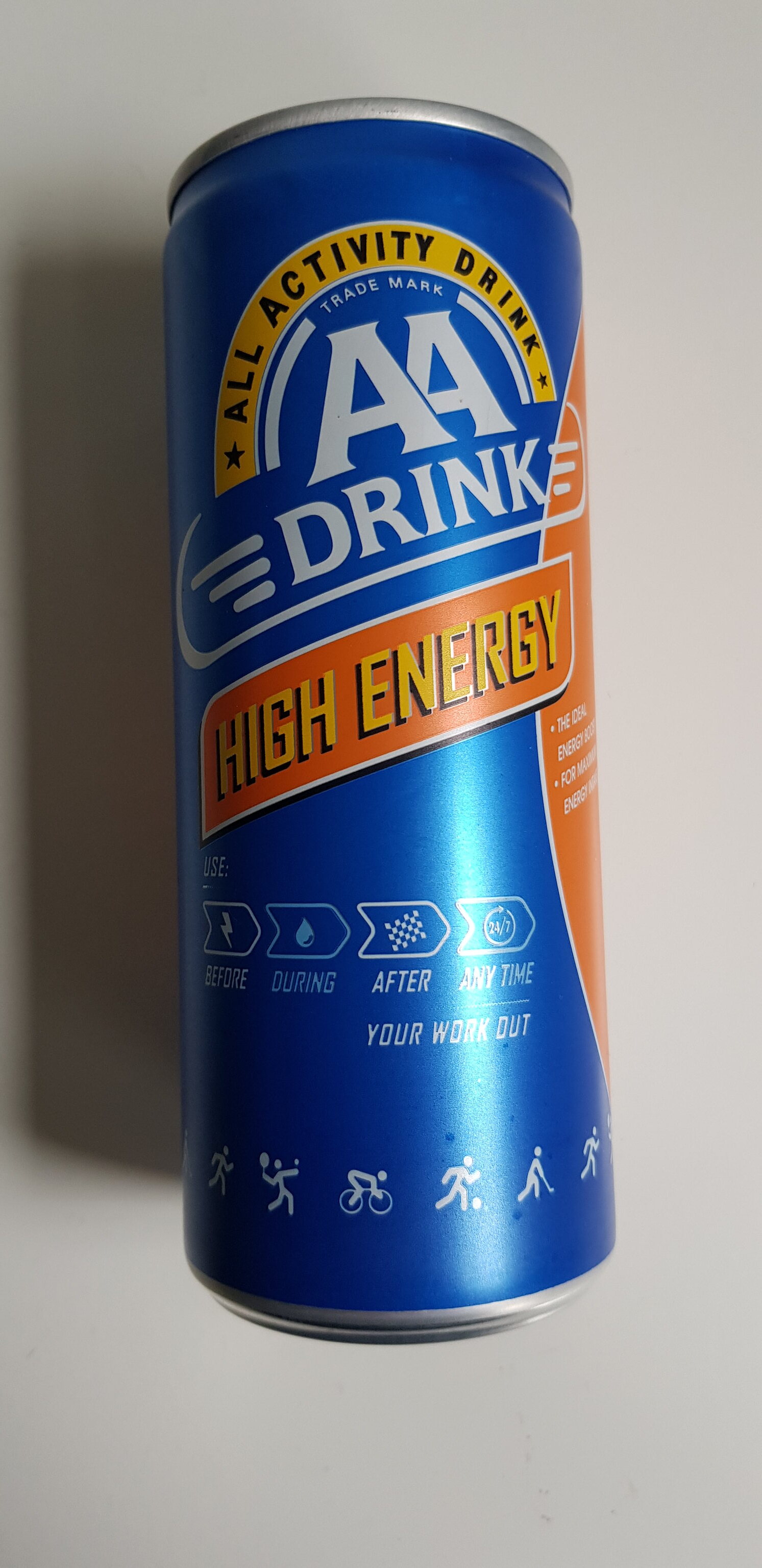Here is a detailed caption for the described image:

"A sleek cobalt blue energy drink can, boasting a satin-like finish, is prominently displayed. The can features a bold, diagonal white text label stretching from the bottom left to the upper right reading 'AA DRINK.' Just below this, there is an eye-catching orange banner with yellow text that declares 'HIGH ENERGY.' Above the 'AA DRINK' label, a semicircular yellow banner showcases the words 'ALL ACTIVITY DRINK.' The bottom section of the can maintains the blue hue, adorned with small, intricate white symbols and text. These include arrows and phrases like 'BEFORE, DURING, AFTER YOUR WORKOUT,' indicating its versatile usage. At the very base, pictograms of various activities such as running, playing tennis, biking, and another unidentified sport emphasize the drink's suitability for an active lifestyle."